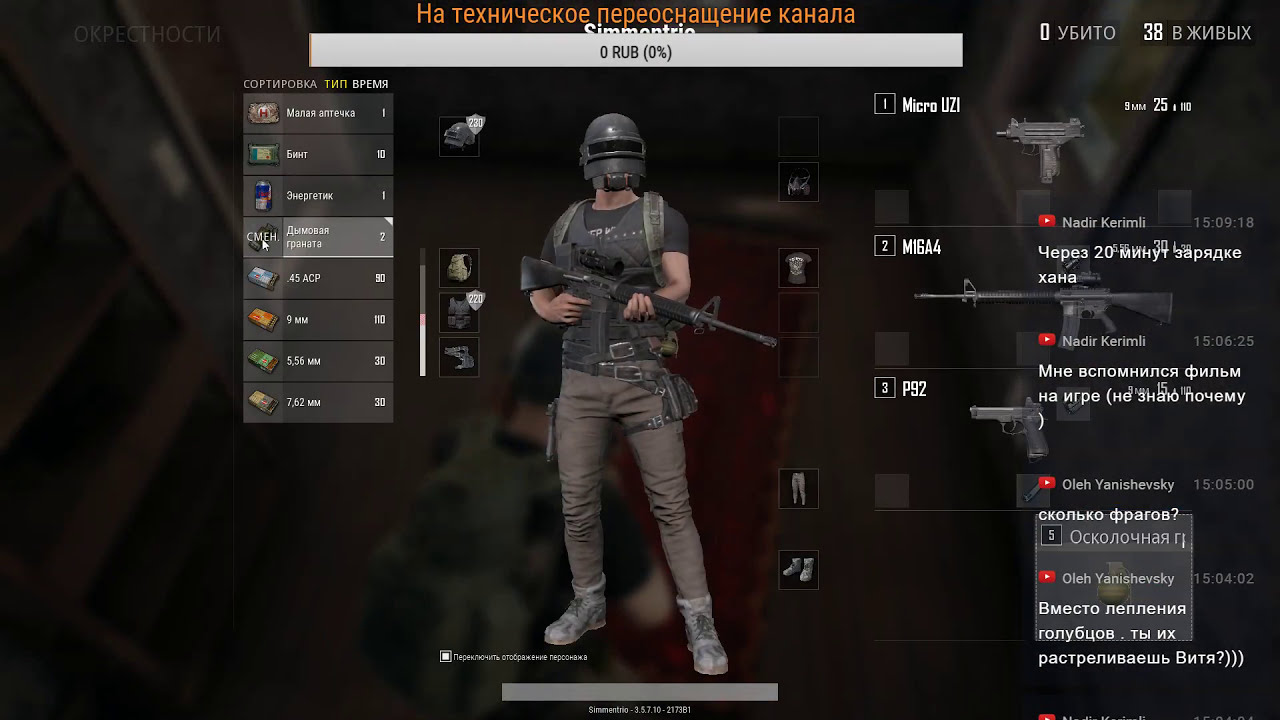The screenshot from the video game, possibly PUBG, showcases a loadout or character customization screen. Dominating the center of the image is the player's character, standing and facing the camera. The character is equipped with a full face welder's helmet featuring a narrow rectangular visor. The neck is exposed, and he wears a black t-shirt under a dark gray utility vest with visible straps from a large gray military-styled backpack. He holds a machine gun, resembling an M16 or possibly an assault rifle, and has a gun holster on his hip. The character is dressed in gray pants tucked into gray boots, which might be described as high-tops. To the right of the character, there is a detailed menu showing various weapons labeled "1", "2", and "3", including an Uzi, an AK-47, and a handgun (P92). This text is slightly superimposed with additional information bubbles. The top of the screen features a gray banner with Russian writing highlighted in orange, stating "zero rub zero percent". On the left, tabs list items the player can acquire. The overall context suggests an inventory management scenario within the game.